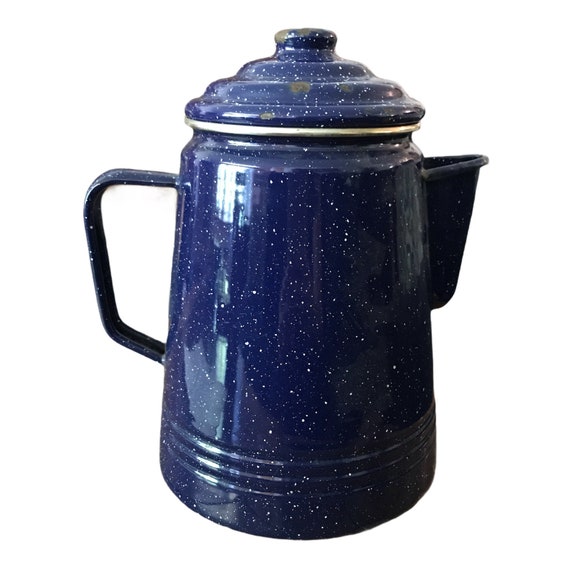This image depicts an old-style, navy blue kettle with white speckled flecks of paint scattered across its surface. The kettle, which appears somewhat worn with chips of paint and scratches, stands tall and cylindrical with a round base that narrows slightly towards the top. It features a large metal handle on the left-hand side and a tall, triangular spout on the right-hand side. The lid, which is adorned with ringed layers that spiral to a smaller cap, sits atop a silver metal ring where it attaches to the kettle. The background of the image is white, which highlights the kettle's reflective surface, suggesting it may be lined or insulated with stainless steel. The reflections captured on the kettle hint at various objects in the room, adding to its vintage and well-used appearance.